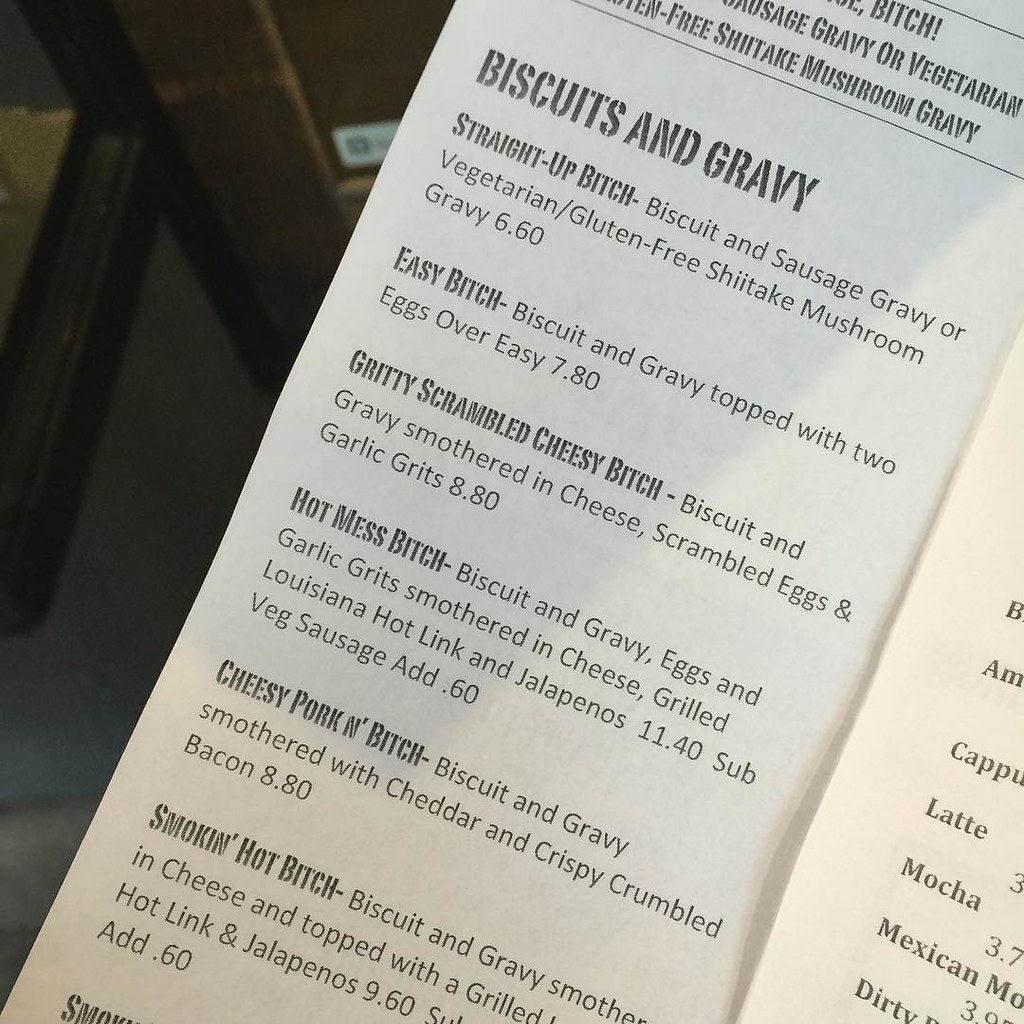This image captures a section of a menu, displayed at a slightly diagonal angle, stretching from the bottom left corner upwards to about a third of the way to the top. Although the top and bottom edges of the menu are cut off, the visible portion reveals a white background with black text. 

Dominating the upper part in the largest font is the heading "Biscuits and Gravy." Beneath this, written in progressively smaller fonts, are the creatively named menu items which include:
1. **Straight Up Bitch**
2. **Easy Bitch**
3. **Gritty Scrambled Cheesy Bitch**
4. **Hot Mess Bitch**
5. **Cheesy Porkin' Bitch**
6. **Smokin' Hot Bitch**

Each name is accompanied by a detailed description of the dish in the smallest font, with prices ranging from $6.60 to $11.40. To the right edge of the menu, a partially visible section lists beverages such as Latte and Mocha, indicating a broader selection of drinks extending off the page.